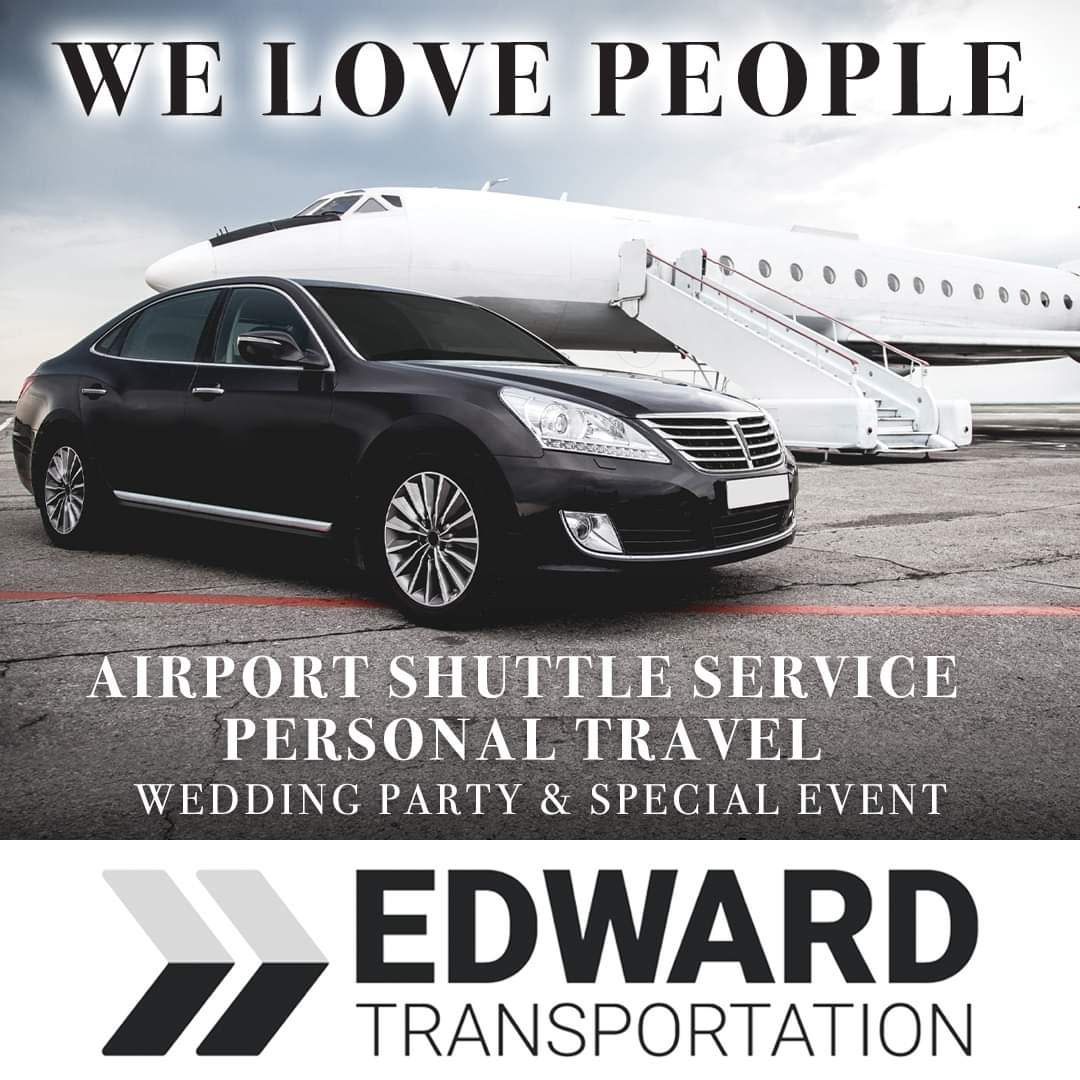This advertisement features a glossy black sedan prominently displayed on a concrete tarmac, marked with a red stripe. The car, a four-door model, faces right and stands before a white private jet positioned in the background. The jet, slightly angled to the left, is equipped with white stairs on its right side leading up to its entrance. The cockpit of the aircraft, visible to the left, features a black rectangle on its nose and four small grey windows above and to the right. Overhead, the sky transitions from dark grey on the left and upper parts to lighter grey in the top right. The top of the image bears the slogan "We Love People" in black text, while the bottom highlights the offerings: "Airport Shuttle Service, Personal Travel, Wedding Party, and Special Event" in white text against the concrete ground. Below the image, on a white background, two chevrons (grey on top and black below) point towards the name "Edward Transportation" in black text.